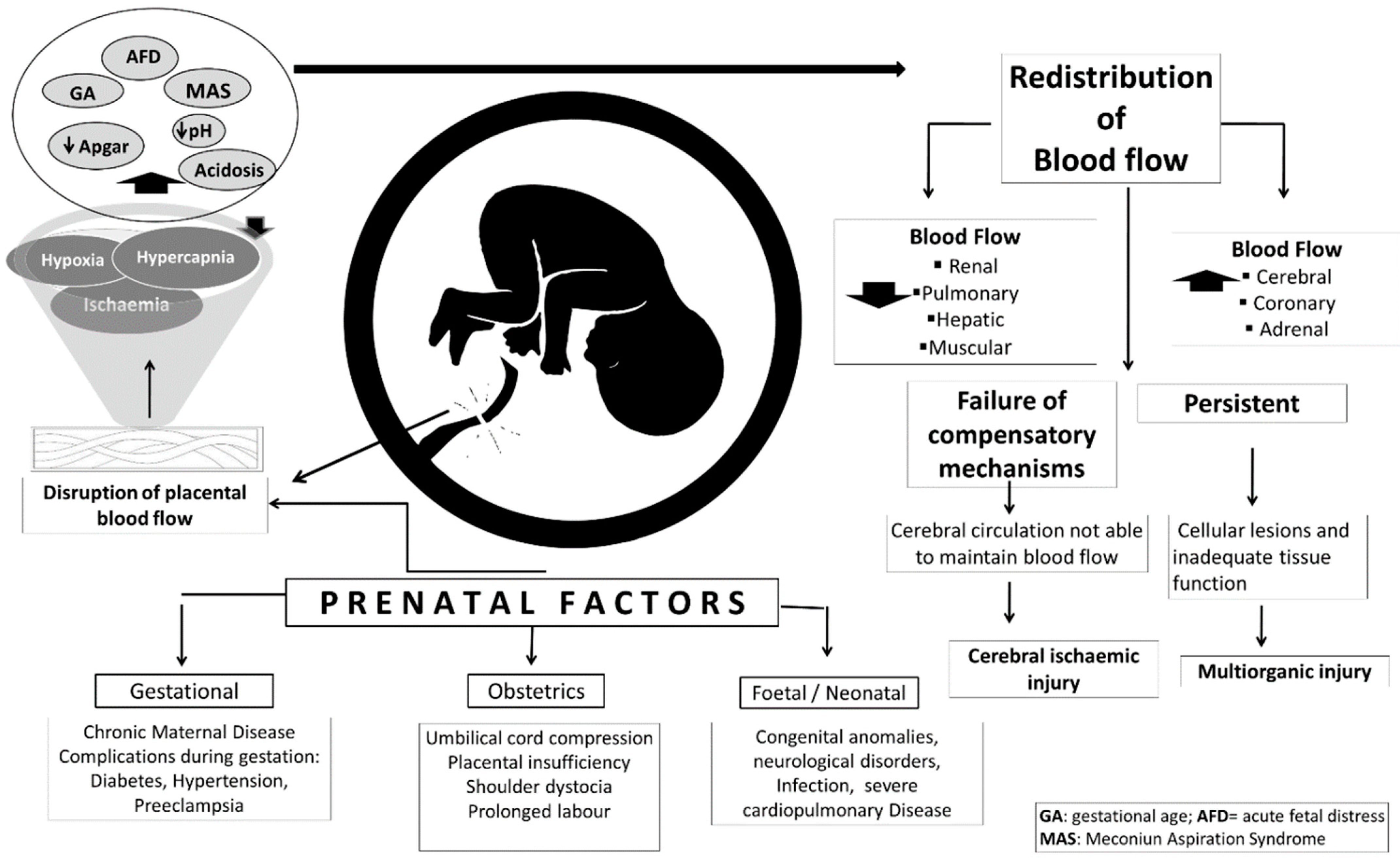This image is an intricate diagram focused on prenatal health, likely sourced from a medical textbook. The chart is centered around a prominently outlined silhouette drawing of a fetus within a thick black circle, located in the center-left portion of the diagram. Directly beneath this illustration is a label titled "Prenatal Factors," which leads to three main sections of a flowchart: gestational, obstetrics, and fetal/neonatal. 

In the upper-left corner, adjacent to the fetal illustration, are several circles labeled with terms such as hypoxia, hypercapnia, ischemia, and abbreviations like GA (gestational age), AFD (acute fetal distress), and MAS (meconium aspiration syndrome). The right half of the image features another flowchart discussing the redistribution of blood flow, with arrows pointing to various types of blood flow in renal, pulmonary, hepatic, muscular, cerebral, coronary, and adrenal systems. 

This section also details potential complications such as failure of compensatory mechanisms, disruptions in cerebral circulation, persistent cellular lesions, inadequate tissue function, multi-organ injury, and cerebral ischemic injury. Additional medical terminology such as placental blood flow disruption, umbilical cord compression, placental insufficiency, and prolonged labor is scattered throughout the diagram. The entire illustration is rendered in black and gray on a white background, emphasizing its scientific and educational purpose.